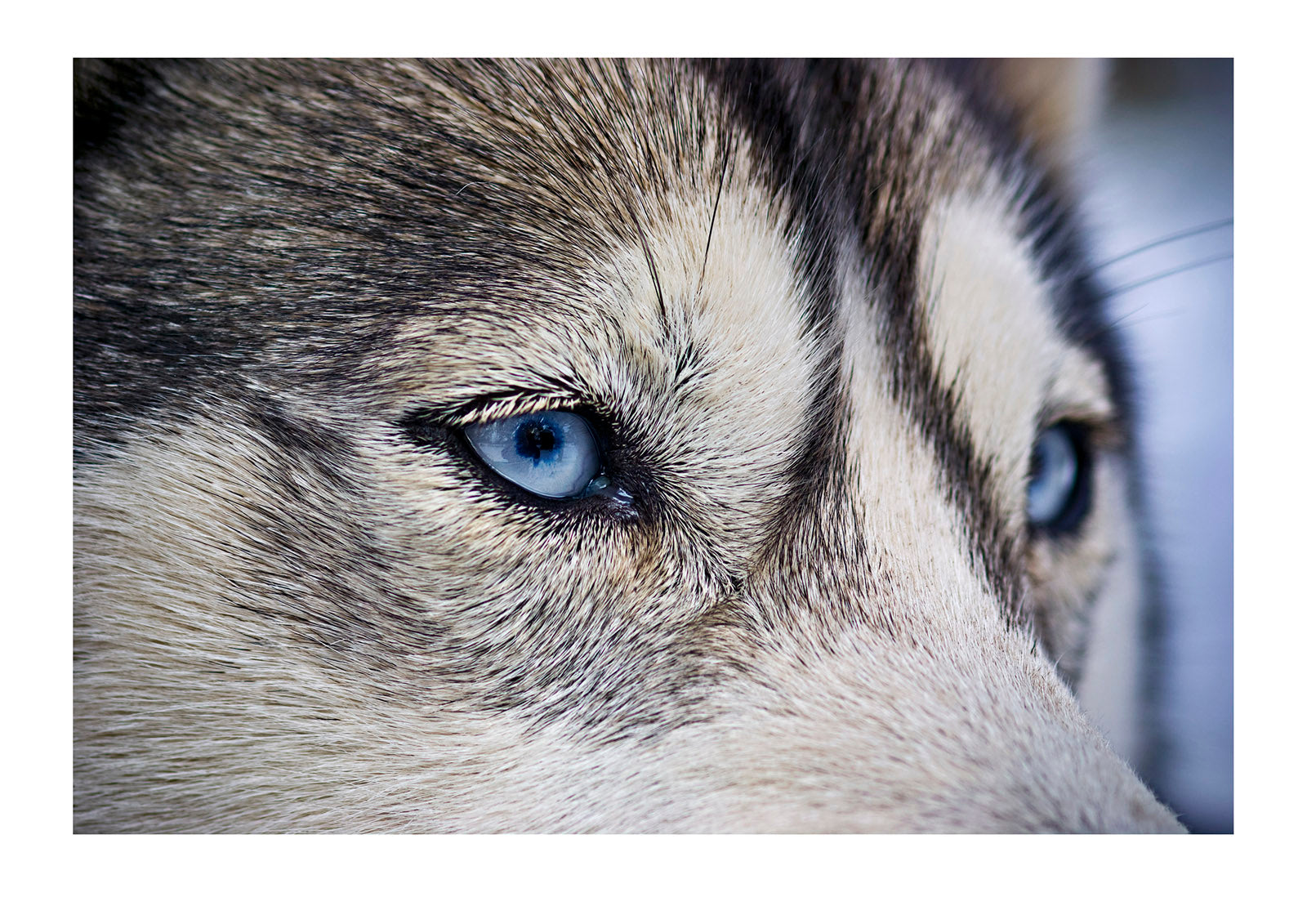A close-up photograph captures the mesmerizing pale blue eyes of a husky. The image focuses on the dog's eyes, which are a strikingly clear blue, contrasted by the dark gray fur on the forehead. Some lighter gray fur is visible just beneath the eyes, emphasizing their brilliance. Whiskers sprout above the eyes, enhancing the dog's expressive gaze. The fur above the eyes mimics the appearance of eyelashes, adding to the captivating look. The photograph does not include the muzzle, nose, or ears, maintaining a tight crop on the eyes and upper face. The background, visible only at the right edge, is out of focus and grayish, providing a subtle backdrop that keeps all attention on the husky's extraordinary eyes. This color photograph contains no text or people, ensuring the viewer's sole focus remains on the dog's stunning blue eyes.